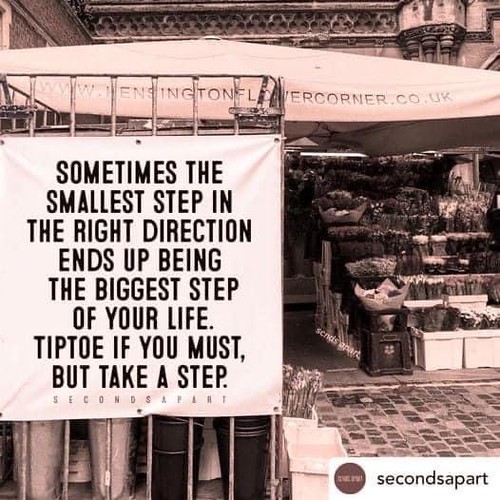This detailed black and white photograph, with a subtle reddish tint, captures an outdoor market scene featuring a charming flower stall. The image’s bottom right corner showcases a brick or stone pavement leading towards a market stall, adorned with a canopy displaying the text "WWW. Kensington Corner Company, UK". The stall is brimming with vibrant floral arrangements, indicating it’s a flower stall. An uplifting banner hangs centered to the left side of the photo, bearing a poignant message in bold black letters against a white background: "Sometimes the smallest step in the right direction ends up being the biggest step of your life. Tiptoe if you must, but take a step." Below this, smaller, faint gray letters mention "seconds apart". The scene is illuminated by daylight, situating the stall in an outdoor setting. A metal fence supports the tent overhead, adding a layer of historic charm to the quaint market atmosphere.